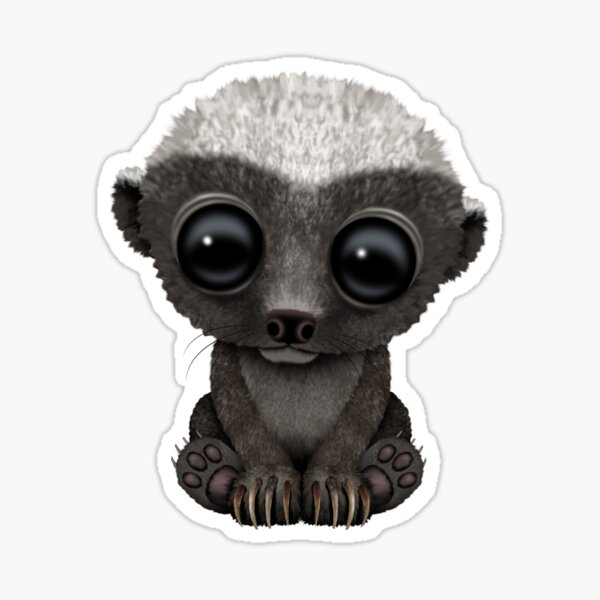The image features a centrally positioned, sticker-like depiction of a marsupial creature on a light gray square background. The creature is outlined by a white border, providing a buffer between the sticker's edge and the character itself. It has an exaggeratedly large head with two strikingly big, round black eyes. The head and parts of its fur are shaded in varying tones of gray, with the top of its head being a notably lighter gray, almost white. The marsupial has a small, brown nose, with lighter gray fur right above it, and dark gray fur covering most of its body. Its chest fur is slightly lighter than the rest. The creature displays long, brown, and light brown claws on its forepaws, which are positioned in front of it as it sits. Its back paws are spread to the sides, showcasing bear-like paw prints with shorter claws. The entire scene has the appearance of being computer-generated.